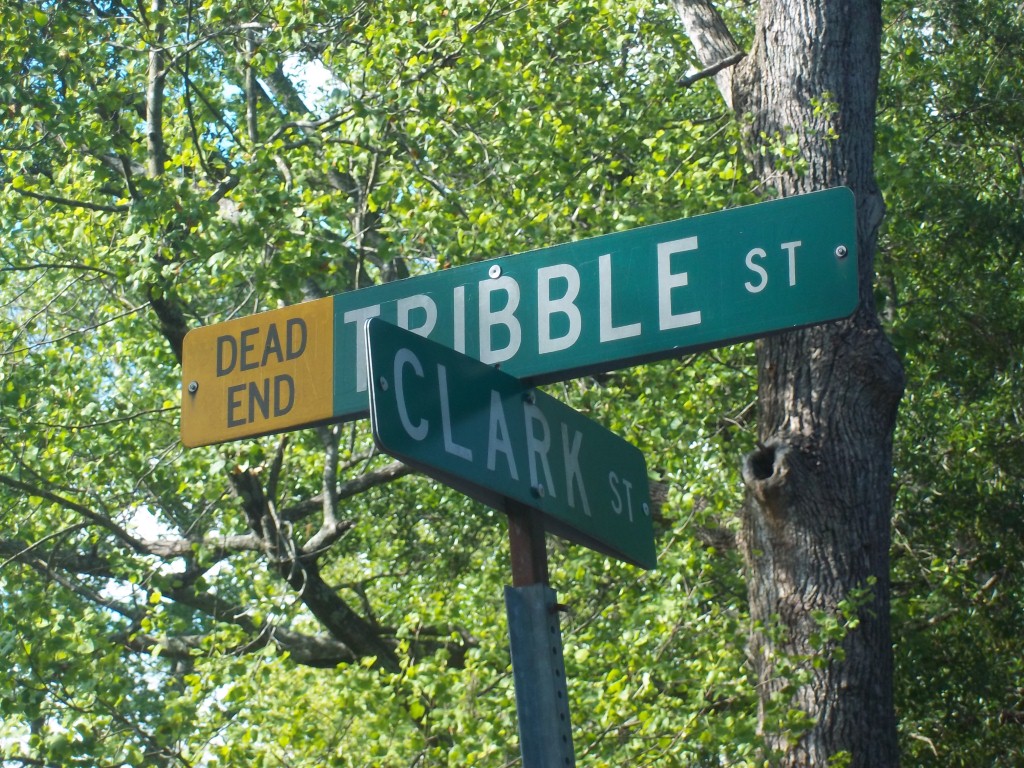This outdoor photograph captures a classic street sign set against a lush, tree-lined backdrop. Dominating the right side of the image, a tall tree rises with its branches and vibrant green leaves extending across the frame, nearly obscuring the blue sky that sporadically peeks through the dense foliage. Emerging from the bottom center of the photo is a pole piercing upwards. At the pole's top, two green street signs are prominently displayed. The lower sign angles slightly downward, reading "Clark Street" in bold white letters. Above it, the second sign is oriented horizontally and face-on, labeled "Tribble Street" also in white. On the left edge of the Tribble Street sign, there is a small yellow section with the black inscription "Dead End," warning of the road's terminus ahead.